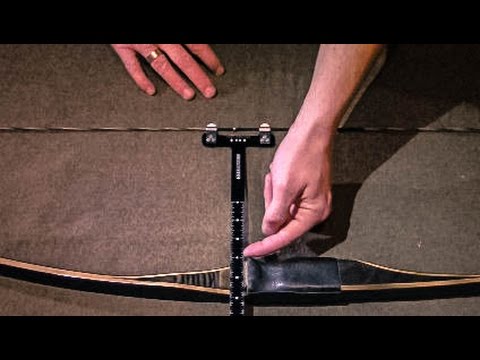The square, full-color photograph, likely taken from an educational video or pamphlet, captures a meticulously posed indoor scene with artificial lighting. There is a distinctive black border along the top and bottom edges with no borders on the sides. The focal point of the image is a wooden archery bow resting on a grayish-brown surface. The bow, complete with its string, showcases a detailed structure that thickens at the handle where an arrow would rest, featuring a black gauge for measuring pull strength.

Entering the frame from the top are two male Caucasian hands. The left hand's fingers are partially visible, prominently displaying a wedding band on the ring finger. The right hand, more fully seen with its forearm, points to a spot on the bow, indicating the black, T-shaped measuring gauge with white markings that lies atop the bow. The gauge appears to be a crucial instructional tool for determining the draw length or pull strength of the bow. The photograph captures the intricate details and positioning, suggesting a precise demonstration related to archery setup or technique.